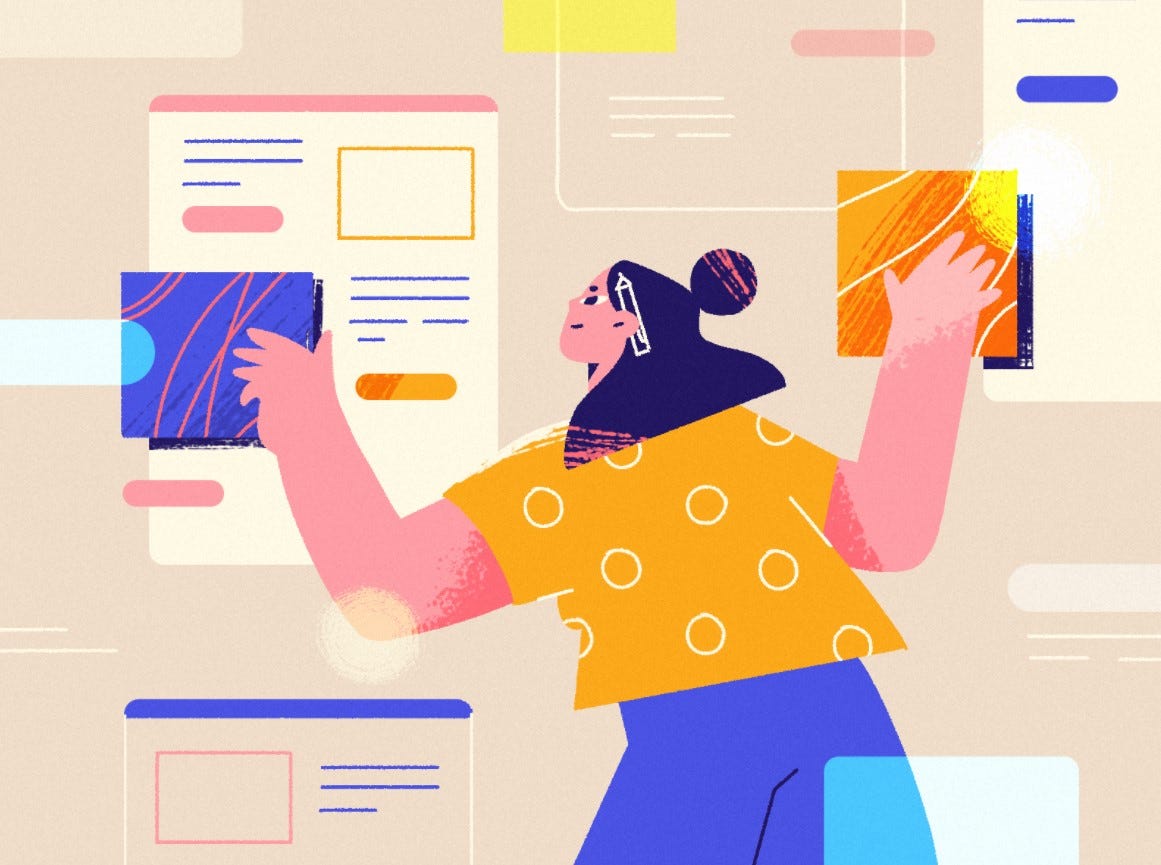This is an illustration of a woman with shoulder-length black hair, styled in a triangular shape with a curve at the top, and a small circular detail on the right. She has a pencil tucked behind her ear and is smiling. The woman is dressed in blue pants and an orange t-shirt with white polka dots. The artwork employs a minimalist style with solid colors and blocky shapes, and the woman has exaggerated features, including overly large hands and arms.

She appears to be interacting with a large vertical sheet, perhaps representing a page she is designing. The page includes a prominent pink bar at the top, blue lines indicating text, and various shapes such as circles and rectangles that likely denote sections and highlights. In her left hand, she holds a blue square with orange lines and a light blue half-circle near the center. Her right hand holds an orange square with white lines and a yellow circle in the top right corner. The woman seems to be arranging these squares on the sheet, which may depict a page of a publication or website. Additionally, a white and pink and yellow box is visible below the squares, possibly a book drop-off. 

Overall, the drawing captures the woman's focused yet cheerful demeanor as she engages in her task.